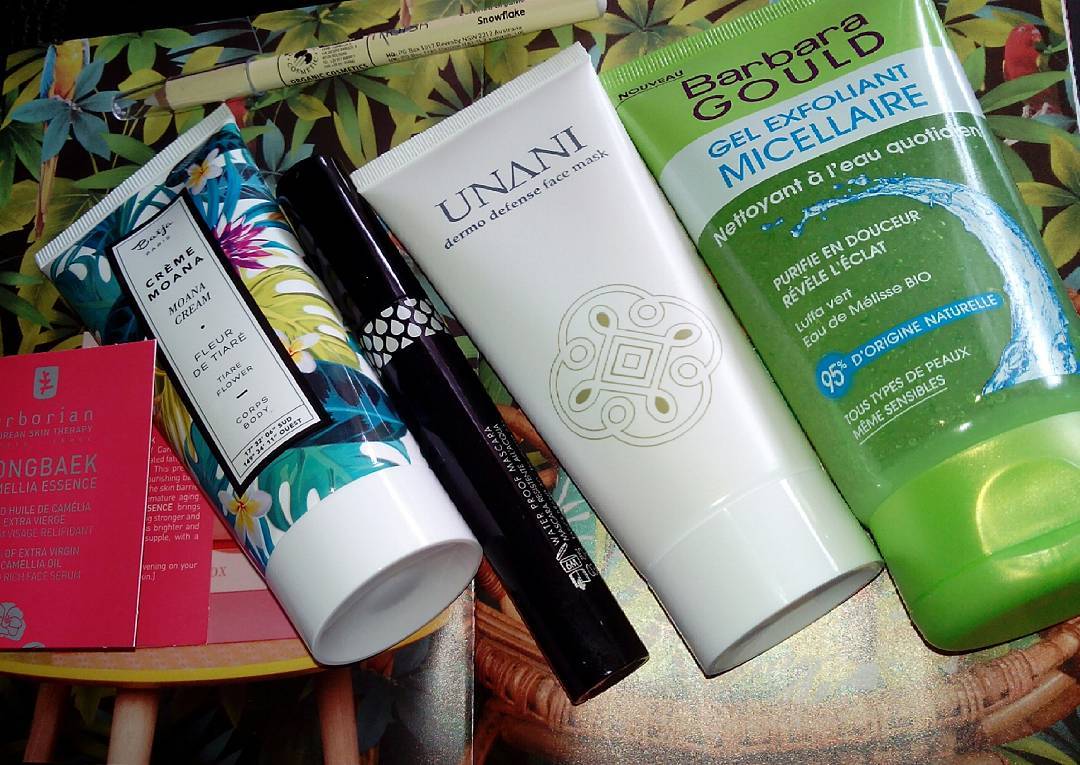The image depicts a neatly arranged lineup of four skincare products, each distinctly branded. From left to right, the first item is a hand cream with simple yet elegant packaging. Next to it is a mascara, followed by another hand cream branded 'Unani.' The fourth item is an Unani Gel Exfoliant, marked by its green packaging and the text 'Micellar Water.' Despite the diversity in product types, all four packages share similar dimensions in terms of length, although they vary in thickness. The backdrop of the image features a printed pattern, providing a visually appealing contrast to the skincare items.